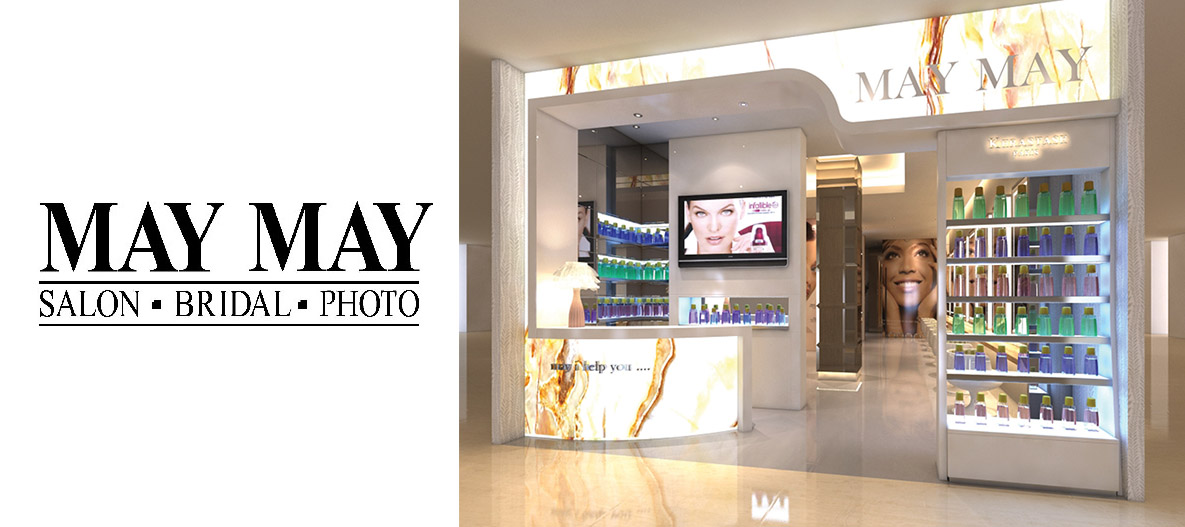The front entrance of "May May Salon.Bridal.Photo" showcases its name prominently on both a sleek grey floor and a bright white illuminated sign with silver letters reading "May May". Underneath the main name, on the left, "Salon.Bridal.Photo" is displayed with distinct red and black lines accentuating the words. The right quadrant reveals the exterior view of the salon, featuring a stylish entrance. To the left of the entrance, a counter is lined with numerous blue bottles, while to the right, colorful shelves display green, orange, and pink bottles. Additionally, there are multiple posters of women's faces visible on the pillars and walls, contributing to the salon's modern and polished aesthetic.